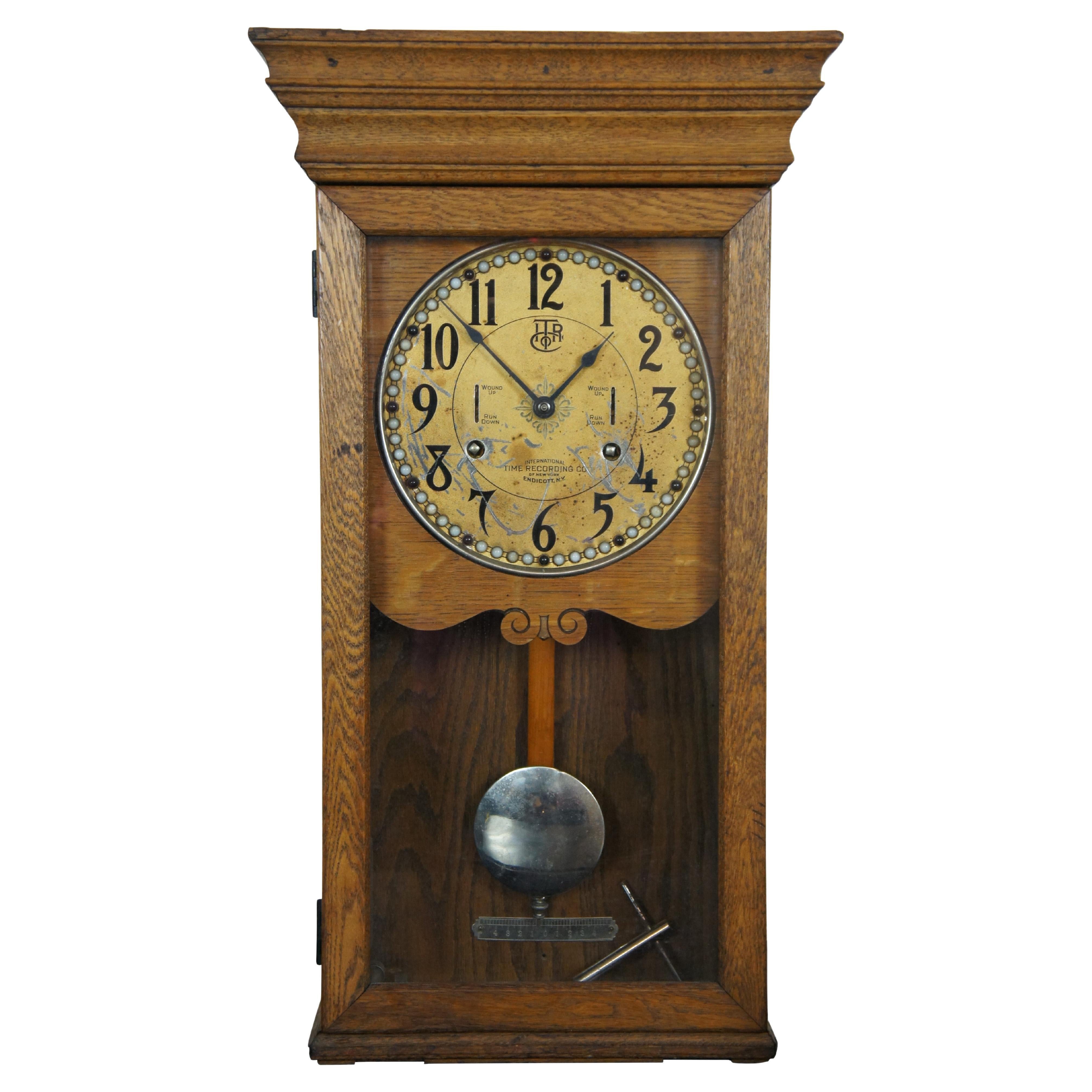This image features a vintage, antique-style clock reminiscent of a grandfather clock, though reduced to about a third of the size. The clock is constructed from medium oak wood that has a light, somewhat aged and worn appearance, further giving it an old and dirty look. The background has been edited out, leaving a stark, textureless white backdrop that accentuates the intricate details of the timepiece.

The clock face, positioned centrally within the wooden structure, has a faded, dingy yellow-beige tone speckled with brown, hinting at its aged nature. Displaying the time at nearly one o'clock, the black numbers from 1 through 12 are prominently visible, each encircled by black beads, adding to the antique aesthetic. Between these, lighter colored beads adorn the positions, creating a unique pattern.

At the bottom of the clock face, the name "Ratchett Indicott, New York" is inscribed, signifying the maker. The clock features long, thin, black hands, slightly out of focus, suggesting movement. Below the main body sits a pendulum, complete with a shiny silver circular attachment and a small ruler. Inside the case, an old key rests just below the pendulum, integral to the clock’s winding mechanism.